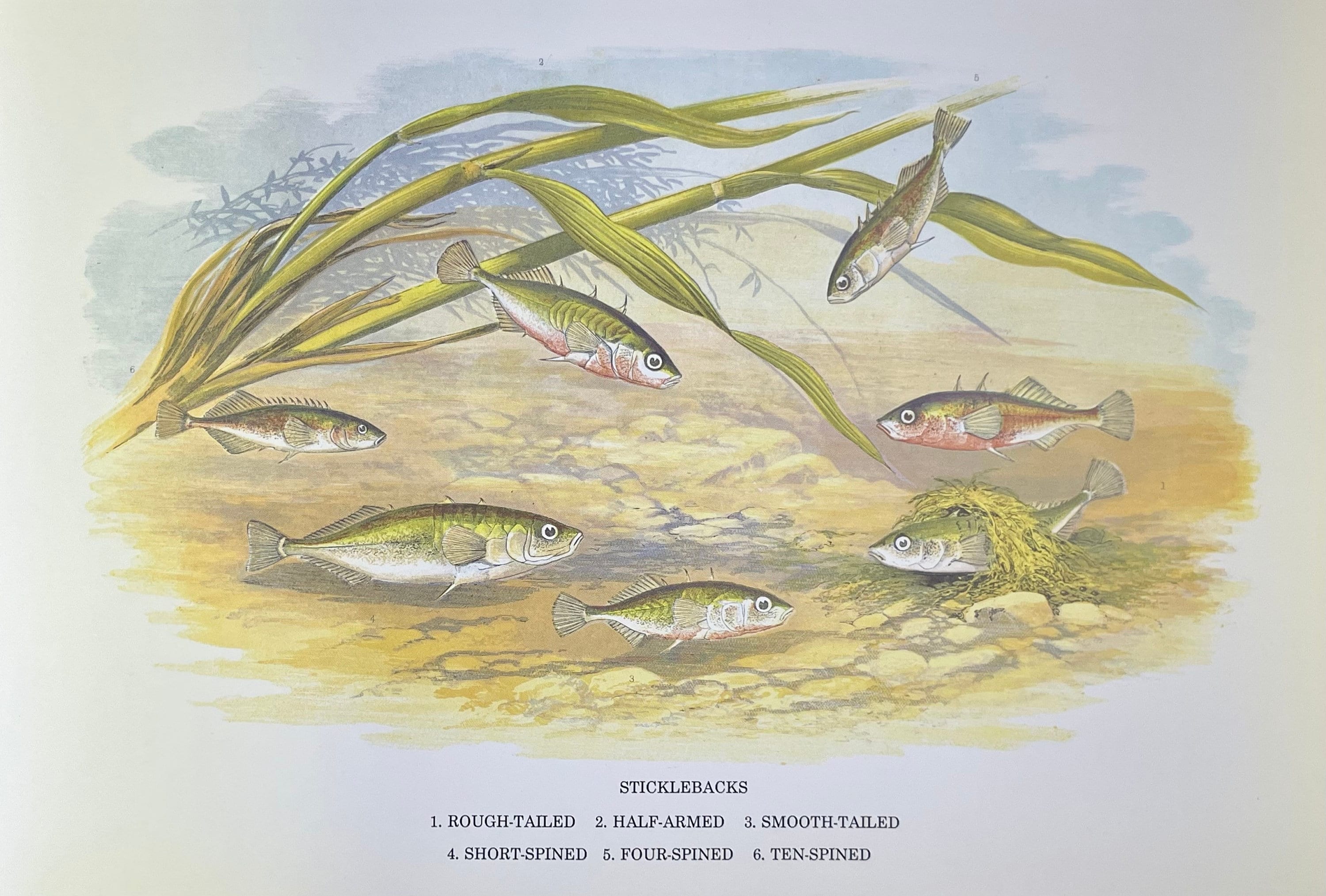The image is a detailed color illustration, likely done in watercolor or oil, of seven small fish, labeled as different types of sticklebacks. The illustration has a landscape orientation with a light gray background and a blue wash across the top half.

In the middle ground, three fish on the left face right while three fish on the right face left, with their profiles clearly visible. The fish at the bottom right is resting on a creamy, textured, sandy surface and appears to be nesting, surrounded by a ring of green moss.

An aquatic plant with long, wavy green leaves extends diagonally from the left side of the image, pointing towards the upper right. This plant contrasts with a gray silhouette of a similar underwater plant behind it.

Each type of stickleback is labeled in black text below the corresponding fish. The labels read: "Sticklebacks: number 1, rough-tailed; number 2, half-armed; number 3, smooth-tailed; number 4, short-spined; number 5, four-spined; number 6, ten-spined."